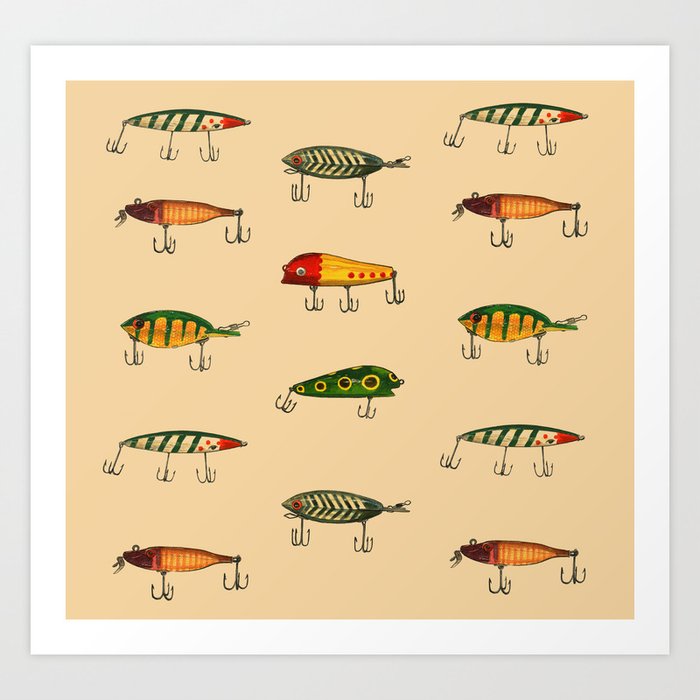The image captures an organized display of fishing lures, arranged meticulously against a square, sherbet orange background enclosed by two borders: a light gray external border and an inner white border. The square image measures roughly six inches by six inches. The fishing lures are positioned in three distinct rows; the left and right rows each contain five lures, while the central row features four. 

These lures, all elongated and narrow like small fish, showcase various hand-painted designs and vivid colors, predominantly featuring vibrant greens. Each lure is equipped with either two or three U-shaped hooks dangling below them, similar to grappling hooks. Among the lures, notable designs include one with a bluegill appearance accented by green stripes, another with a red head and a yellow body marked by three red dots, and a lure with black stripes and a red head. The top left lure is particularly distinctive with its green-striped, white-bodied design and red markings, reminiscent of an eye. Overall, the detailed and colorful array is indicative of handcrafted care and precision aimed at attracting various types of fish.